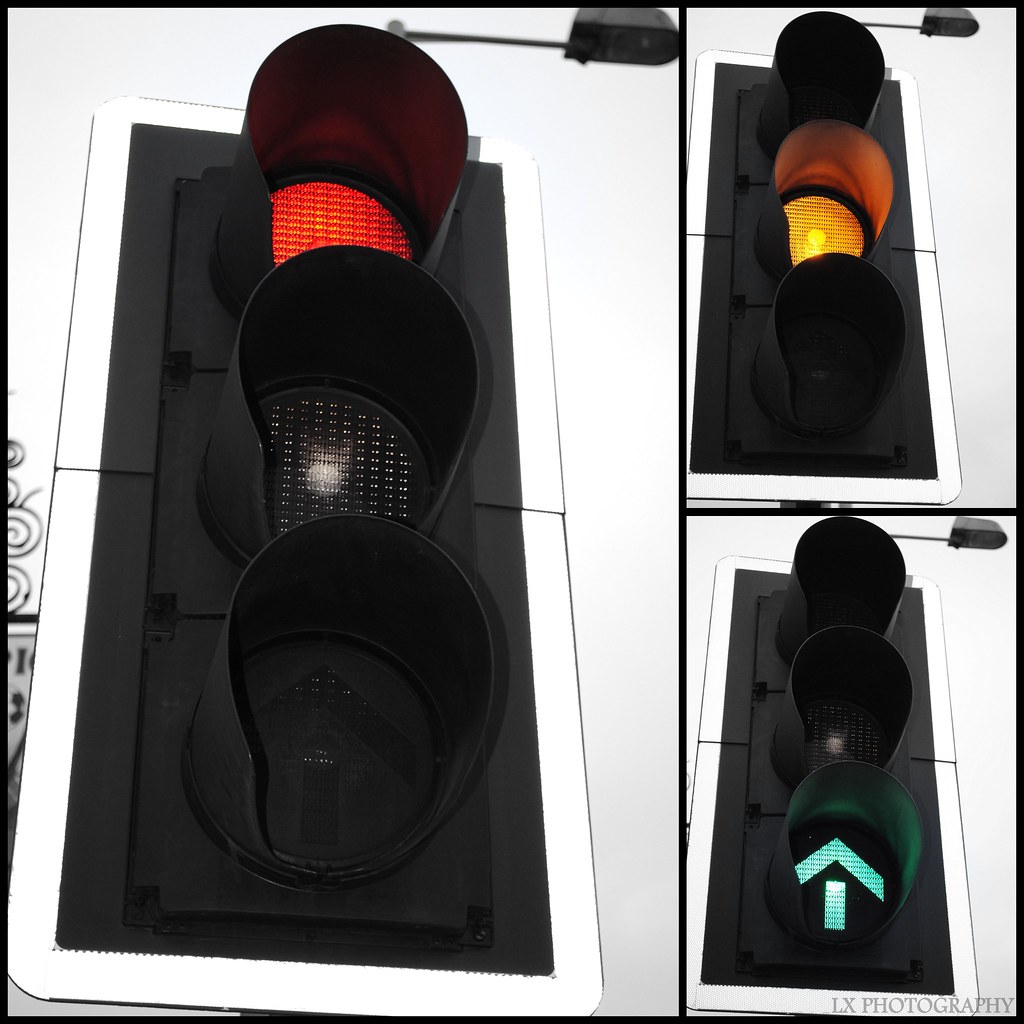This artistic image features three close-up photographs of a stoplight, meticulously captured with professional photography techniques, as evidenced by the clear and detailed imagery. The primary focus is on the largest image on the left, showcasing a black stoplight with its red light illuminated at the top, while the middle and bottom lights remain unlit. The bottom light also has an unlit arrow pointing upwards. The stoplight is framed in a circular black frame, set against a wider rectangular black background with a white border. The upper right section of the composition displays the same stoplight with the yellow middle light glowing, and the other two lights unlit. The lower right section features the green bottom light with an illuminated upward-pointing arrow, while the other lights are not lit. The backdrop of the image reveals a light white sky suggesting a cloudy morning, along with a black, unlit streetlight. A photographer's watermark reading "Alex Photography" is subtly placed in the bottom right corner.